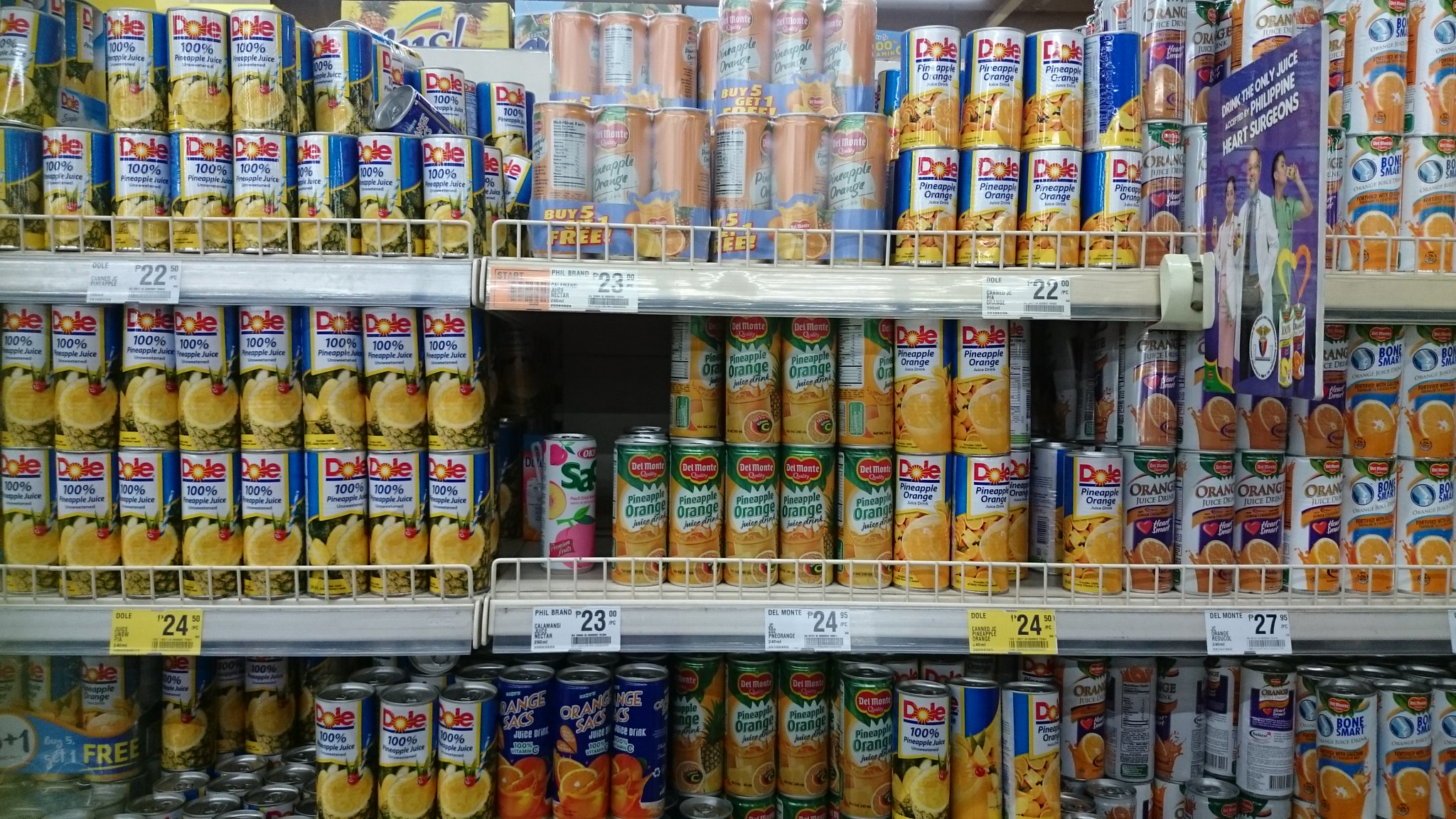This image features a selection of Dole fruit cans prominently displayed on a grocery store shelf. The Dole cans, characterized by their narrow and tall shape, feature dull red lettering on a white background at the top of each can. The display spans three shelves, with the cans neatly lined up, showcasing mostly pineapple varieties along with some other fruits. Despite the small size of the text on the Dole cans, the brand's dominance on the shelves is evident. Adjacent to the Dole display is a competitor brand with indistinct blue writing and an orange image on the front of the cans. The Dole prices are clearly visible, ranging from 23 to 24 cents, while the competitor's prices are slightly higher, at 27 cents. The shelves themselves are white, set within the context of a typical grocery store aisle.